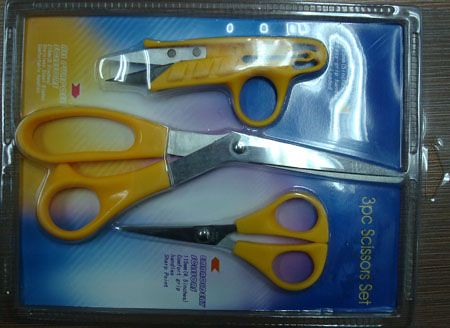In this detailed image, we observe a three-piece scissor set encased in a clear plastic package. The set comprises two pairs of scissors and a unique snipping tool, all featuring yellow handles. The main pair of scissors, positioned centrally, has long silver blades and an extended yellow grip area. Flanking it are a smaller pair of scissors, approximately four inches long, and a distinctive yellow-handled tool resembling a pocket knife with two sharp silver tips. The packaging includes a blue, white, and yellow paper backdrop with partially legible information. Clearly displayed in yellow text on the bottom right corner are the words "three-piece scissor set." The entire package rests on a wooden table with visible dark brown streaks, noticeable on the right side of the image.